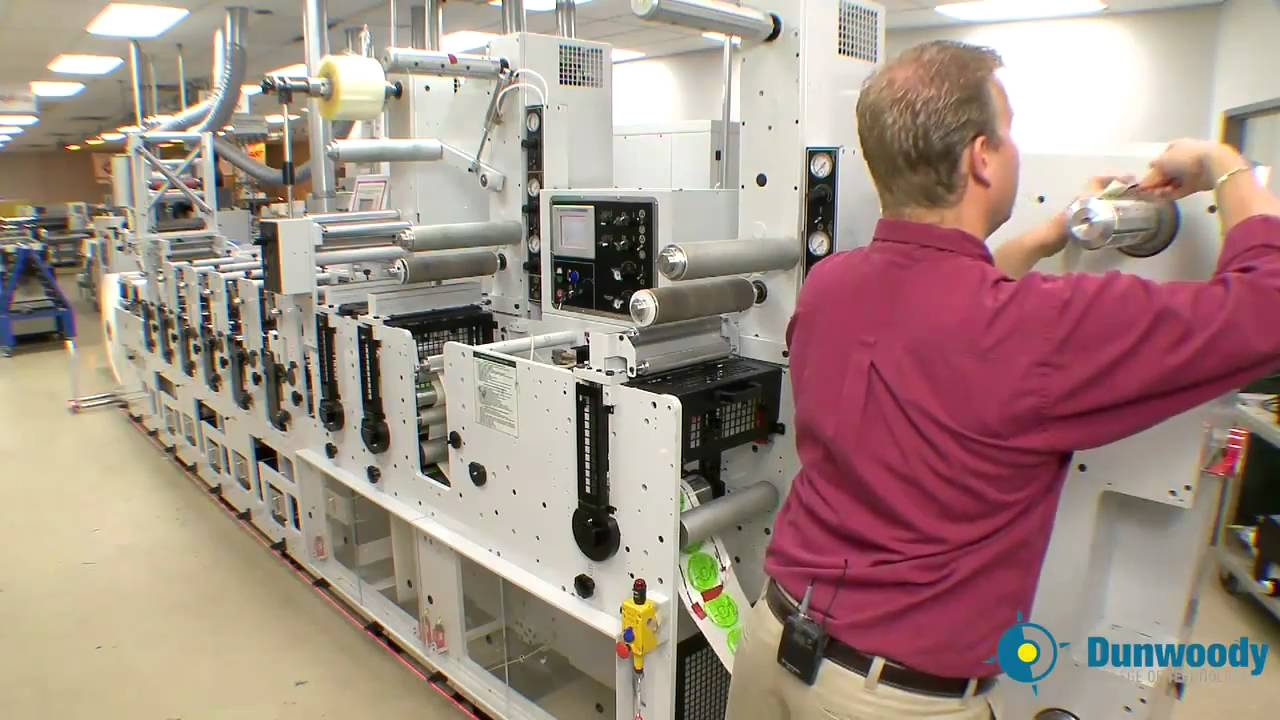In this detailed photo taken inside a brightly lit room with low ceiling tiles, a middle-aged Caucasian man is seen from the back, working on a large mechanical device. The man has medium blonde, slicked-back hair with a noticeable bald spot and is wearing a maroon, long-sleeved collared shirt tucked into khaki chino pants, secured with a black leather belt. A walkie-talkie or similar black device is clipped to the back of his belt, and he also wears a bracelet on his hand. The machinery in front of him appears to be a massive printing press or similar industrial device, characterized by off-white and black panels with numerous silver-gray rollers. There is a visible black panel with knobs, and various steel poles extend from the device. The room, likely a factory or workshop, has a beige floor, and the mechanical device features a logo that includes the word "Dunwoody" in blue, alongside a bullseye symbol. To the left, another extensive white machine can be seen, with rollers and a section dispensing a white sheet with green stickers, resembling a labeling or tape application mechanism.